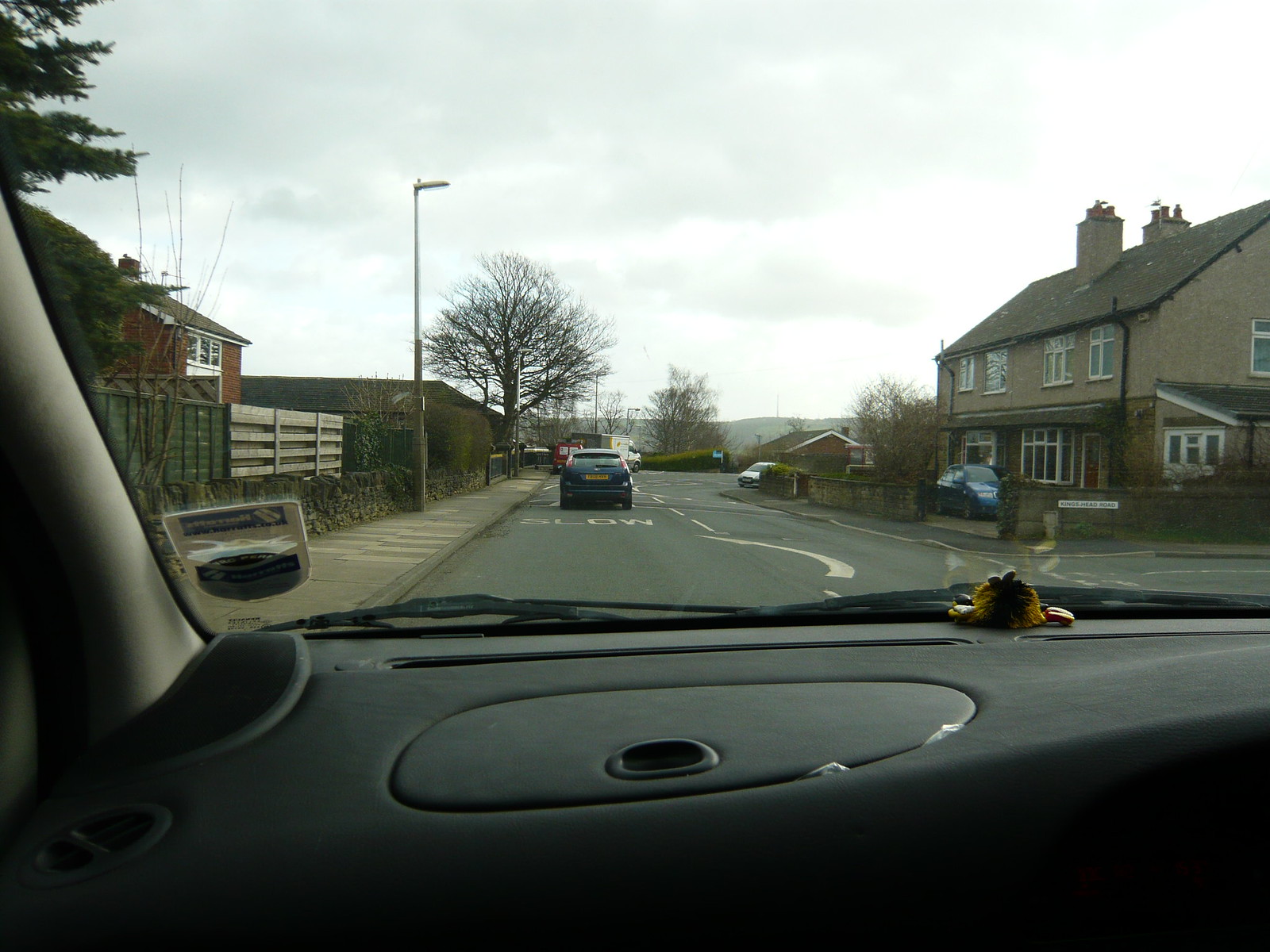The photograph captures the view from the left-hand front seat of a right-hand drive car, suggesting a European setting, likely in the UK. Through the windshield, the car's wipers are visible, aligning with the passenger side airbag blowout panel, indicative of its right-hand steering configuration. The car is traveling on a two-lane asphalt road, occupying the left lane, consistent with driving norms in countries like England.

Ahead, a small blue car is noticeable, bearing a wide, yellow European-style license plate. The road surface displays the word "SLOW," signaling an upcoming right-hand curve. Flanking the road, single-family dwellings are discernible. On the left side, a tall fence obscures much of one house. On the right, a house enclosed by a short brick or cement fence features stucco walls adorned with numerous windows and white trim. A car is parked at the front, within a small entryway, completing the scene.